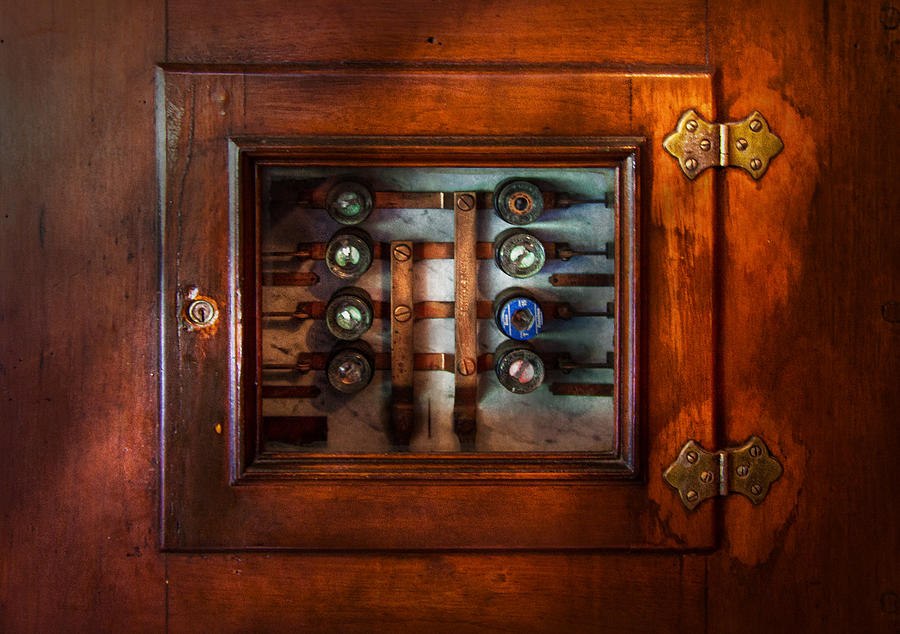This image depicts an antique, likely Victorian-era, fuse box situated on a wall of dark, aged wood. The square-shaped door of the fuse box, crafted from the same dark wood, features a clear glass panel in its center, allowing a view of the intricate components inside. Prominent within the glass panel are eight fuses, four on the left and four on the right, accompanied by brownish, possibly copper, bus bars beneath each fuse. The wood wall and the door show signs of wear, with lighter areas notably around the two ornate hinges on the right side, which seem to be handmade and secured with six screws (three per side of each hinge). The door also has a small keyhole on the left side. The colors visible within the image include various shades of brown from the wood, brass-like hues from the fuse components, as well as hints of orange, blue, gray, white, and black from the background and the electrical elements inside. The overall composition, with its central door and visible mechanisms, gives the impression of a mechanical and meticulously crafted historical artifact.